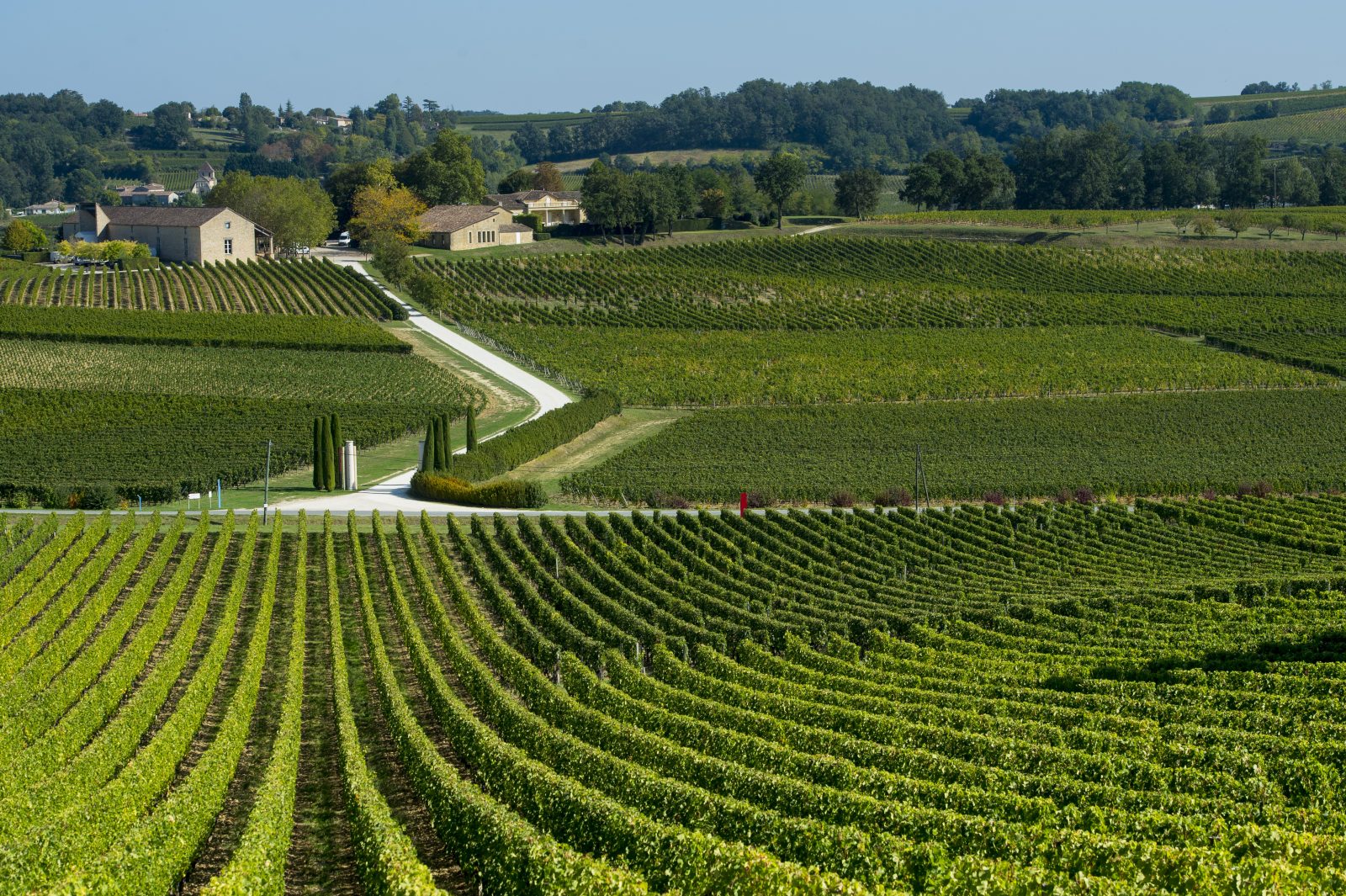The image captures an immaculate and organized farm, featuring perfectly aligned rows of grapevines in the foreground, their meticulous arrangement devoid of any stray leaves. The farm's pristine layout is accentuated by a white road that extends towards beige-colored farm buildings, including a large barn with a triangular roof, a house, and possibly another structure. The buildings are framed by dark green trees in the backdrop and a clear blue sky that speaks of daytime tranquility. Along both sides of the road are additional sections of farmland, each with plants in various stages of growth, creating a neat and combed-over appearance. The fields are divided into different sections with another road running horizontally in the middle, and a grassy area separating the sections, enhancing the overall organized aesthetic of the farm.